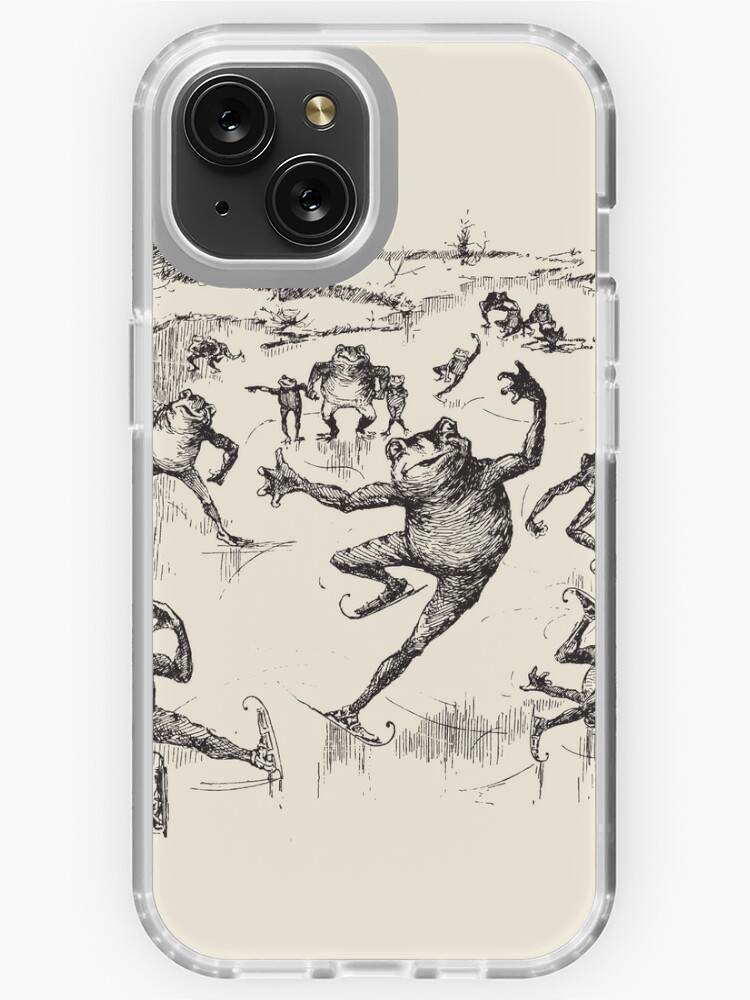The photograph showcases the back of an iPhone with a custom black-and-white backplate, featuring intricately designed frogs ice skating. The phone itself has a distinct camera layout, with two giant lenses diagonally opposite each other—one in the top left and the other in the bottom right—along with a small round metallic element in the top right and a miniature hole in the bottom left. The case is clear around the edges, allowing an unobstructed view of the whimsical artwork and the phone's unique camera features.

The illustrated scene on the backplate depicts several frogs gliding gracefully on a frozen lake, surrounded by a snowy bank. At the center of the image, a prominent frog strikes an animated pose with both hands up and one leg extended while balancing on the ice. Around him, other frogs join in the merriment. Notably, a frog just behind him appears to be walking rather than skating, holding hands with two smaller frogs, who point excitedly as if on a joyful vacation trip. The overall design captures a lively and heartwarming winter activity, harmoniously blending human-like behaviors with the charm of frogs enjoying an ice-skating adventure.